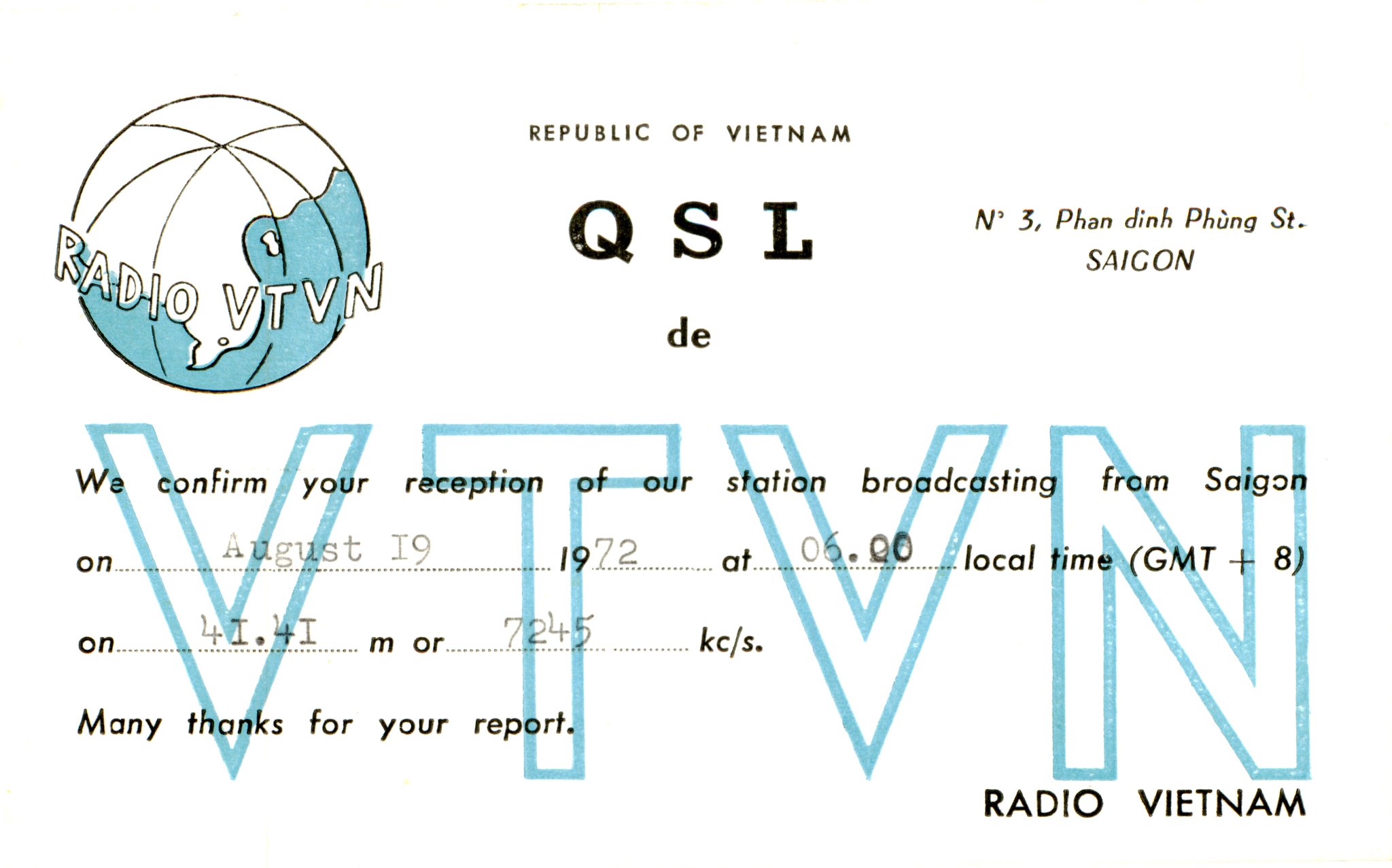The image features an old QSL receipt from the Republic of Vietnam prominently displaying the logo of Radio VTVN in the upper left corner. This logo includes a globe with light blue-green landmasses and the text "Radio VTVN" in white capital letters, appearing as if it’s orbiting the globe. The top one-third of the document is marked by text reading "Republic of Vietnam," followed by "QSL" and "Day," and the address "Number 3, Phan Dinh Phuong Street, Saigon." The bulk of the document confirms the reception of a signal received from Radio Vietnam broadcasting from Saigon on a specified date. The date "August 19th, 1972," and time "05:00 local time, GMT +8" are typed in, indicating the receipt's purpose. The words "We confirm your reception of our station broadcasting from Saigon" are superimposed over the large letters "VTVN" that occupy the lower two-thirds of the document. At the bottom right, "Radio Vietnam" is inscribed in black letters. A note at the bottom thanks the recipient for their report.